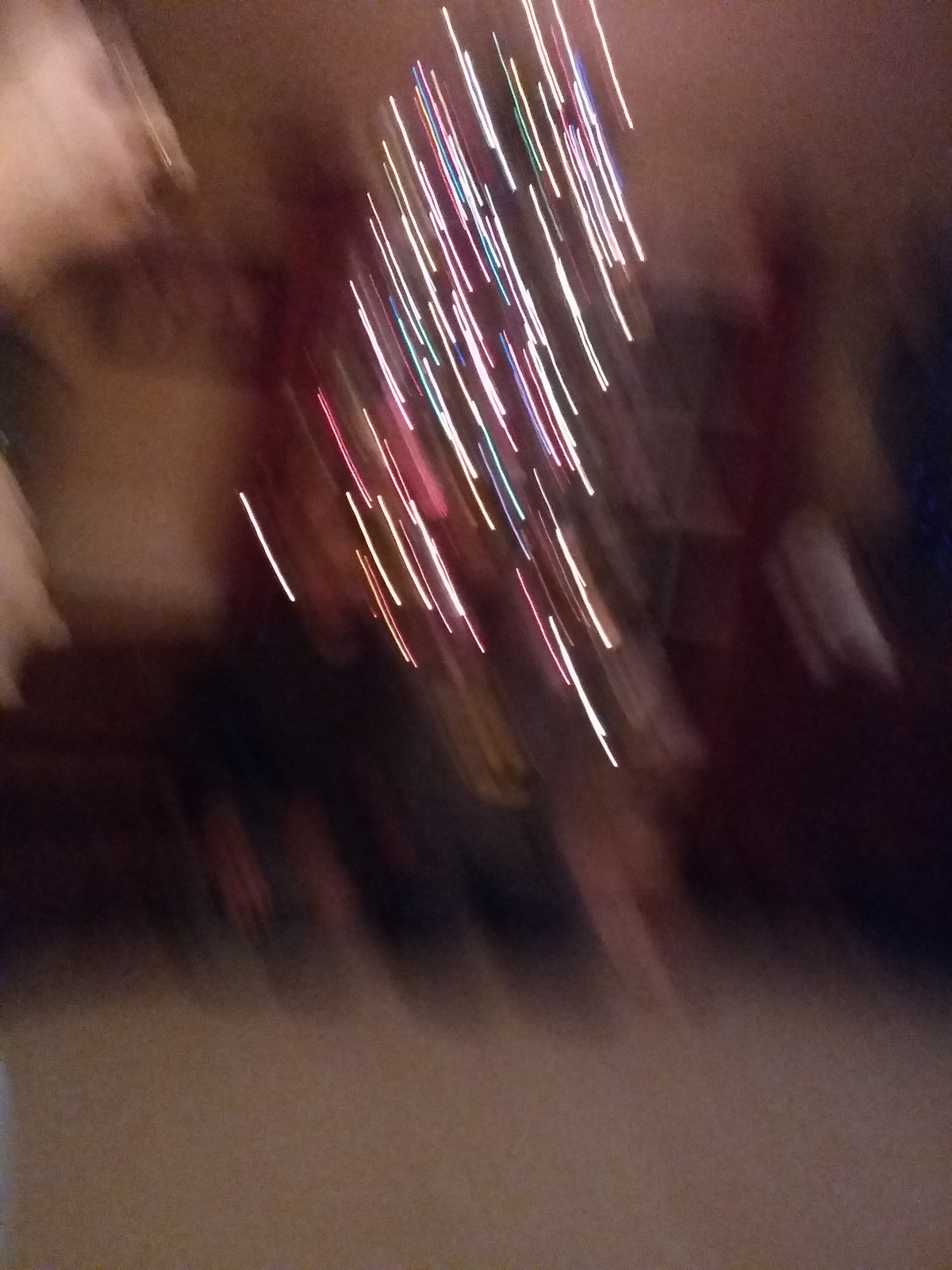The image is an extremely blurry photograph taken indoors, possibly in a house or apartment. The overall scene is out of focus, making it challenging to discern specific objects. The background appears to feature a dark setting with minimal natural lighting, possibly illuminated by lamps. In the middle of the image, there's a cluster of colorful lights, including pink, orange, white, purple, blue, and green, appearing as elongated, vertical streaks, suggesting the lights were captured in motion. Behind these lights, there may be a shoe rack with some cubbies holding shoes and others empty. On the ground, two pairs of shoes are somewhat identifiable: one gray pair with pink shoelaces and a black pair. The surrounding area includes indistinct shapes and colors, hinting at additional objects and possible furniture, but their details are obscured by the blurriness of the image.